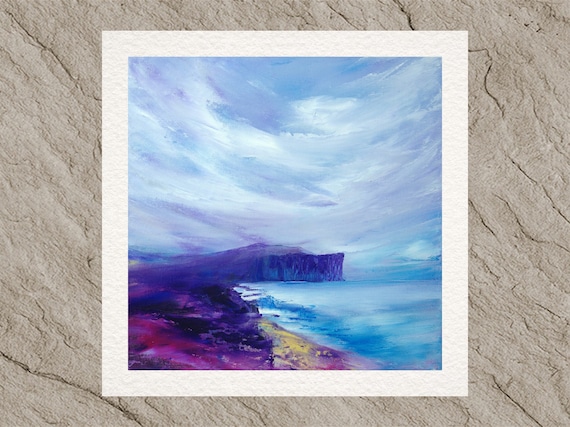This image captures a vibrant painting of a picturesque shoreline, displayed against a textured, weathered wooden surface marred with age. Nestled within a white border, the painting vividly portrays a dynamic scene where a cliff or peninsula, tinged in shades of purple, juts dramatically into the blue and white waters on the lower right. The left side of the painting suggests a colorful shore, adorned with red, yellow, and dark blue accents that evoke a floral landscape. Above, the sky is a canvas of swooping brushstrokes with hues of white, purple, and blue, simulating clouds drifting across a serene blue expanse. The overall composition is framed in a simple, possibly digital white mat, adding to the depth and contrast of the multicolored artistic piece.